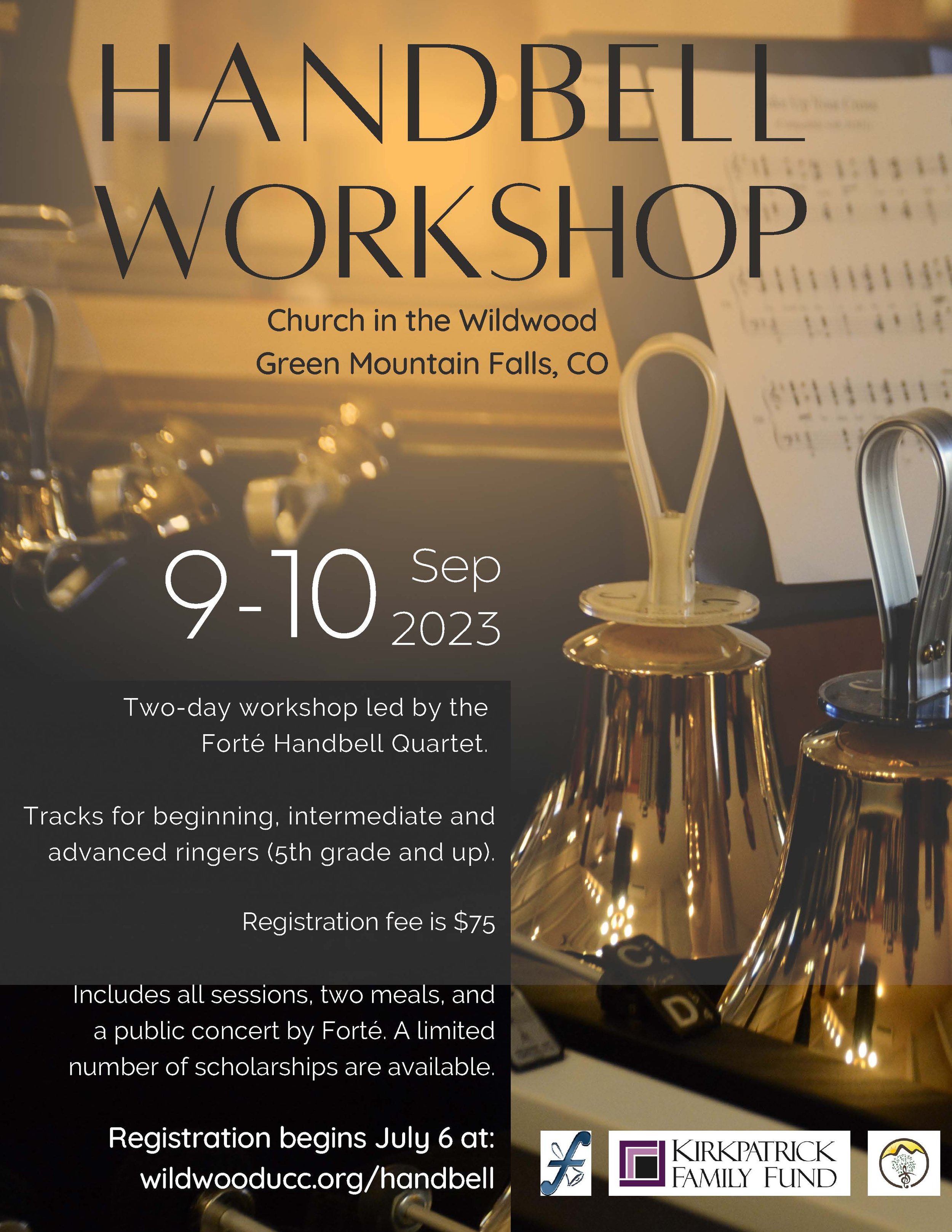The flyer is an announcement for a Handbell Workshop, featuring a sophisticated and somewhat dark color palette primarily comprised of blacks and grays, with goldish hues adorning the top. At the very top, in bold black capital letters, the flyer prominently displays "HANDBELL WORKSHOP." Directly below, in a smaller font, it states the location: "Church in the Wildwood, Green Mountain Falls, Colorado."

The bottom half of the flyer on the left-hand side is densely packed with printed information, including the dates "9-10 SEP 2023" and a description of a two-day workshop led by the renowned Forte Handbell Quartet. It highlights that there are tracks available for beginner, intermediate, and advanced ringers, specifically targeting participants from fifth grade and up. The registration fee is listed as $75, covering all sessions, two meals, and a public concert by Forte. It also mentions the availability of a limited number of scholarships. Registration details are provided, with a starting date of July 6th and the URL "wildwooducc.org/handbell."

On the right side of the flyer, there are three logos: the leftmost, resembling an F note with a flute intersecting it diagonally; the middle one labeled "Kirkpatrick Family Fund"; and the rightmost, an enigmatic circle.

The background imagery includes several handbells, with two prominently displayed on the right, as well as a snippet of sheet music visible in the top right-hand corner. Additional handbells are scattered subtly in the background, complementing the overall dark tones and gold accents of the flyer.